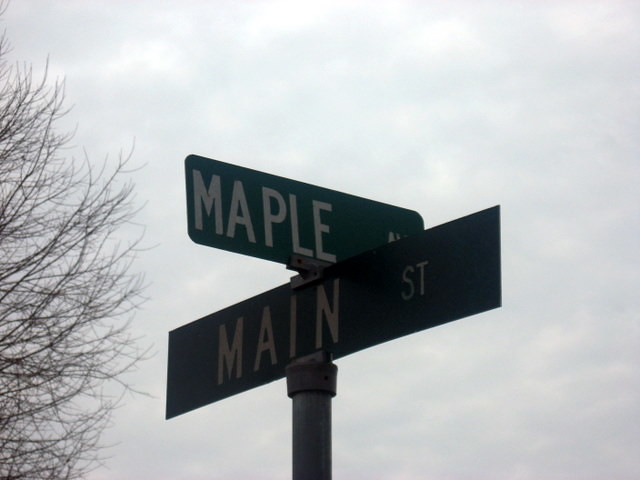This close-up photograph captures a slightly rectangular, landscape view of the intersection at Maple Street and Main Street. The image is taken from a ground-level perspective looking upward, showcasing the street signs attached to a black pole. The signs themselves are a dark green color, juxtaposed against an overcast sky filled with light gray clouds. On the left side of the photo, a leafless tree with dark brown branches stands starkly, hinting at the winter season.